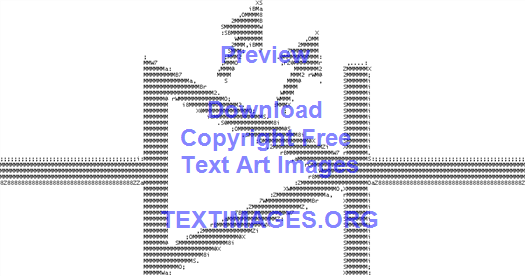The image features a text art design against a white background, composed of alternating black characters. The primary structure in the center resembles an electronic symbol for an LED, consisting of a horizontal line attached to a right-pointing triangle, with the triangle's point intersected by a vertical line. This line extends vertically upwards, forming a cross-like shape at the triangle's apex. Additionally, two filled arrows branch off at a 45-degree angle towards the northeast from the top of the triangle. Above these arrows, in purple text, the word "Preview" is displayed, followed by "Download" directly below. Further down are the phrases "Copyright Free" and "Text Art Images" on subsequent lines. At the bottom, the source "TEXTIMAGES.ORG" is prominently featured in capital letters. The entire design is meticulously crafted using various standard characters and letters, showcasing a blend of artistic and electronic schematic elements.